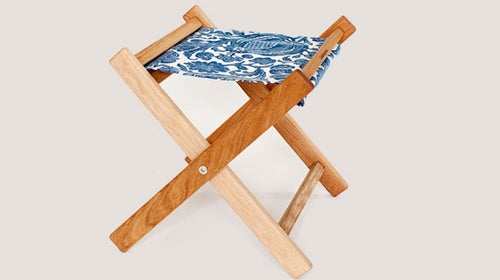The image features a portable, foldable stool with a cantilever design, characterized by its X-shaped wooden frame when open. The stool's wooden structure comprises multiple slats, varying in stain from dark brown to a much lighter tone, enhancing its multicolored appearance. These wood pieces are connected by simple hinges, allowing the stool to collapse and unfold easily. Across the top of the X-shaped frame stretches a piece of fabric serving as the seat, which is secured by the wooden slats. This fabric boasts a quilted-like design with a floral pattern in shades of blue and white. The image, oriented horizontally and taken from a front-side view, has a plain white background, highlighting the stool’s distinct features and portable, practical design.